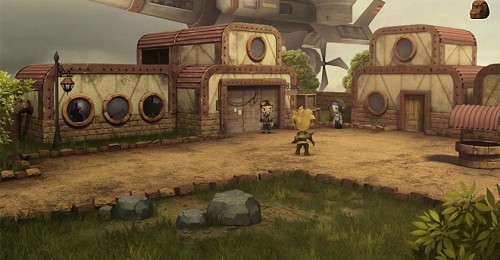In the foreground of this gameplay capture, lush green grass and a vibrant green bush are visible, adjacent to a sandy dirt area with a tan hue. A green, human-like figure with blonde hair stands on the earthy terrain, gazing intently towards two other figures near a set of brown and tan houses characterized by porthole-style windows with golden frames. One of the houses has an old-fashioned street lamp positioned nearby. In front of the homes, a brown human-like figure, dressed in brown clothing, and a gray human-like figure, dressed in gray clothing, can be seen. In the background, part of an airship with a tan coloration is visible, adding a hint of adventure to the scene.